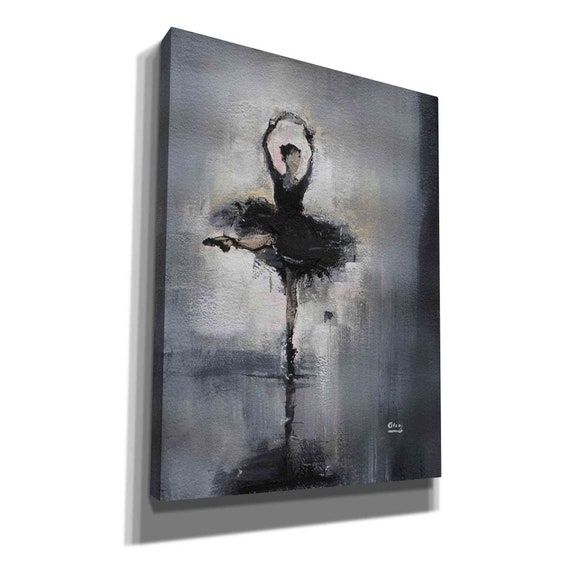The image depicts an abstract, three-dimensional canvas that stands out with its thick square profile. This modern artwork, set against a plain white wall, features a striking combination of neutral tones, including black, white, gray, and a touch of light brown. A noticeable element is the white scrawled signature in the bottom right-hand corner, adding a personal touch to the piece. 

The focal point of the painting is an abstract representation of a woman's silhouette, evoking the image of a ballerina. The figure is portrayed with both hands raised above her head, arms locked together, and one leg pointed and extended gracefully to the side, suggesting a mid-spin dance movement. She is adorned in a dark gray or black long-sleeve dress with a voluminous skirt. The background is a compelling mix of black, white, and varying shades of gray, which melds and contrasts dynamically with the figure.

This expertly photographed artwork appears to be hand-painted and could easily be perceived as a professional's piece, inviting viewers to infer their own meanings and emotions. The drop shadows cast on the wall add depth and dimensionality, enriching the visual experience of this captivating abstract modern art.